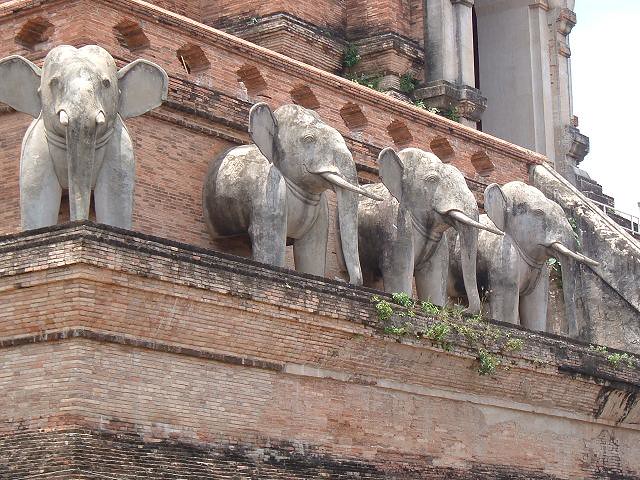The image captures the side of an old, worn brick structure, featuring four grey stone elephant statues that appear to be materializing halfway through the façade. Positioned on a ledge, these elephants display prominent tusks and long trunks. Their bodies seem to emerge only halfway from the building, with just their heads, front legs, and partial torsos visible, while their hind sections are absent. The light orange or rustic red color of the brick contrasts sharply with the grey stone of the elephants, emphasizing their presence. The building’s architectural style hints at an Asian influence, possibly reminiscent of a temple. Adding to the scene are signs of age and wear, including some greenery like vines and an overall faded appearance. The elephants, positioned as though guarding the building, lend a sentinel-like quality to the structure. Additionally, the image features a brick railing with diamond-shaped cutouts above the elephants and a white column doorway, further detailing the architecture of this ancient structure.